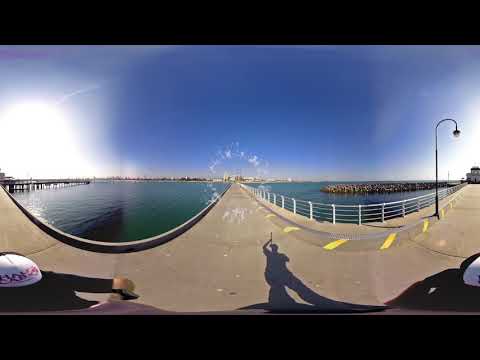In this panoramic image, we observe a view that stretches across a pier leading out into a vast body of water, under a clear blue sky with minimal clouds. The pier is paved with concrete and features a yellow stripe running along its right side, while a white railing guards its edge. The image appears to be taken from the perspective of a standing man, whose shadow is visible at the foreground, suggesting it's taken outdoors in the middle of the day. On either side of the pier, we can see two individuals wearing hats, positioning them against the man in the center.

The water flanks both sides of the pier, and in the distance, a cityscape rises on the far shore. Visible on the right is a large stone rock wall extending into the water, and at its terminus, we see a substantial white building. On the left, there's a sizable dock supported by wooden stilts.

Dominating the center of the image is a unique visual feature: a white, circular mark resembling thin clouds, which adds a distinctive touch to the scene. This image, characterized by its fisheye lens effect, displays slight curvature and stitch marks from the merged photos, creating a sweeping, slightly curved view of the picturesque setting. The sun is positioned to the left, bathing the entire scene in natural light, enhancing the mix of colors that include black, blue, purple, white, gray, green, and yellow. The overall effect presents a vibrant, detailed snapshot of a serene, pier-side landscape between city and sea.